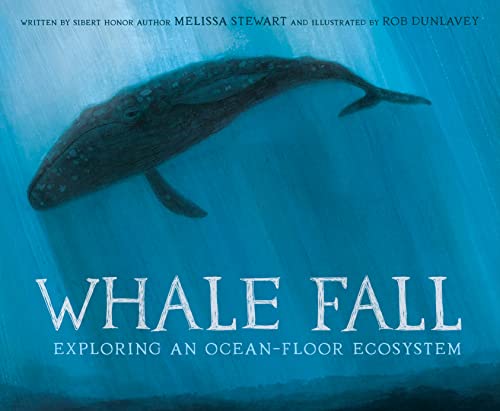The image appears to be a book cover set against a blue background, resembling either a painting or a slightly blurry photograph. Dominating the center is a dark whale, almost black, viewed from above and heading towards the ocean floor. The whale's tail extends to the upper right, and a fin juts out toward the lower center, emphasizing its large, dark presence in the water. At the top of the image, in small black font, it says, "Written by Sibert Honor author Melissa Stewart and illustrated by Rob Dunlavy." Near the bottom, in bold white letters, the title reads, "Whale Fall," with a subtitle below in light blue letters, "Exploring an Ocean Floor Ecosystem." This cover conveys a detailed, immersive look into the marine world, focusing on the ecosystem where whales live out their lives.